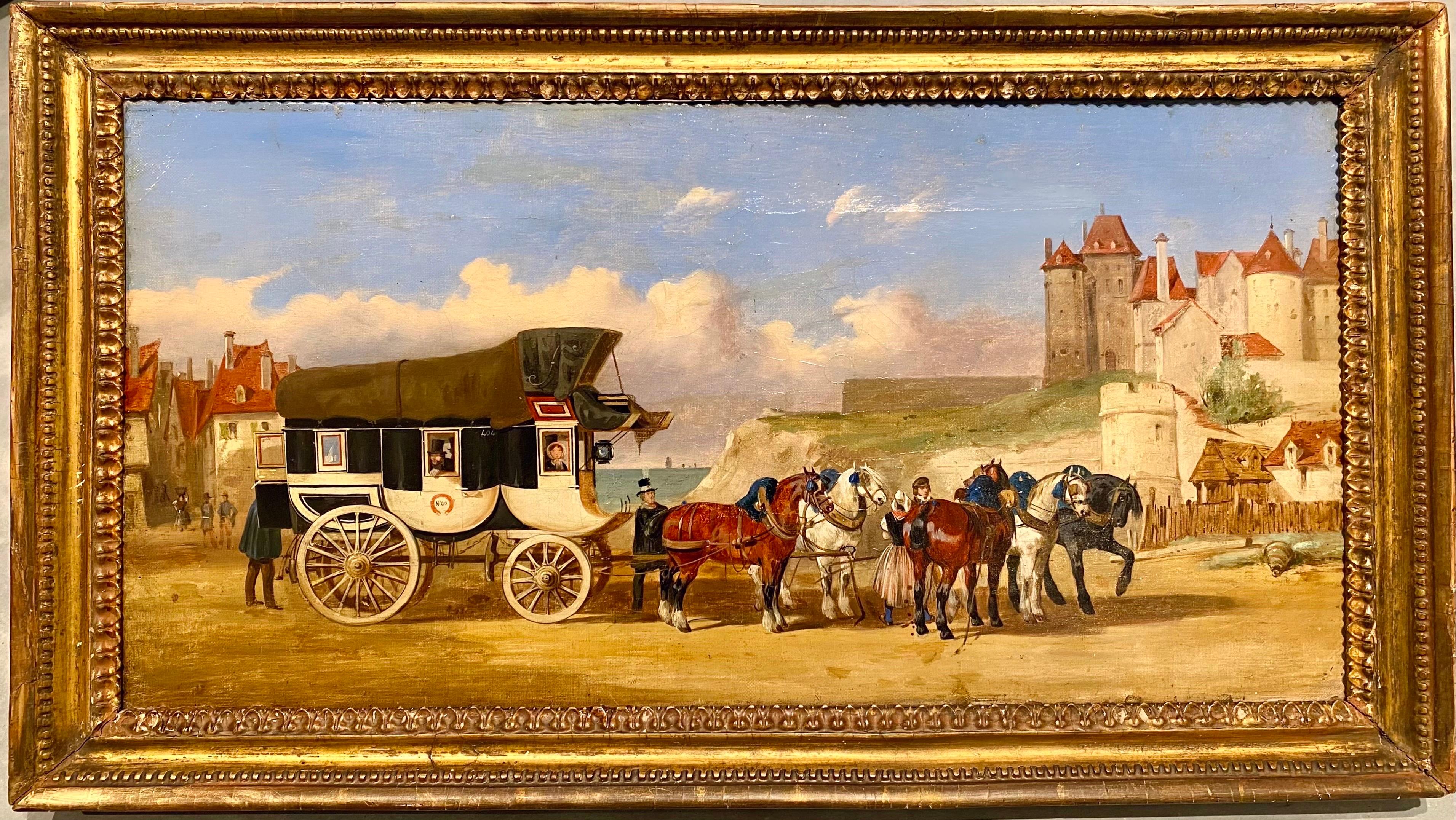The image is a highly detailed oil painting from the 18th century, presented in a beautifully ornate wooden frame painted in a gilded gold hue. The scene captures an intricately designed horse-drawn carriage, complete with a curved chassis and side windows. The carriage, topped with a gray-brown canvas, is positioned outdoors in a bustling setting. To the left, there is a quaint village with distinct red rooftops, while to the right, on an elevated hilltop, stands a structure reminiscent of a castle.

At the center of the composition is a small body of water, adding depth to the scene. The carriage is pulled by a team of six horses, displaying a variety of colors - from tannish orange and reddish hues, to pure white and black ones. The most prominent horse, a reddish one with black legs and white-tipped hooves, is harnessed nearest to the carriage.

The painting also includes several figures: a young lady seated at the front of the carriage, a mature gentleman in the middle, and another individual standing at the back with the door open, possibly retrieving luggage. Additionally, a coachman is positioned behind the horses, while a gentleman and a lady stand in between them. A person in a long gray coat and brown pants can also be seen at the very back of the wagon. The sky suggests it’s either daytime or early evening, with clouds visible in the distance, adding to the painting's atmospheric quality.